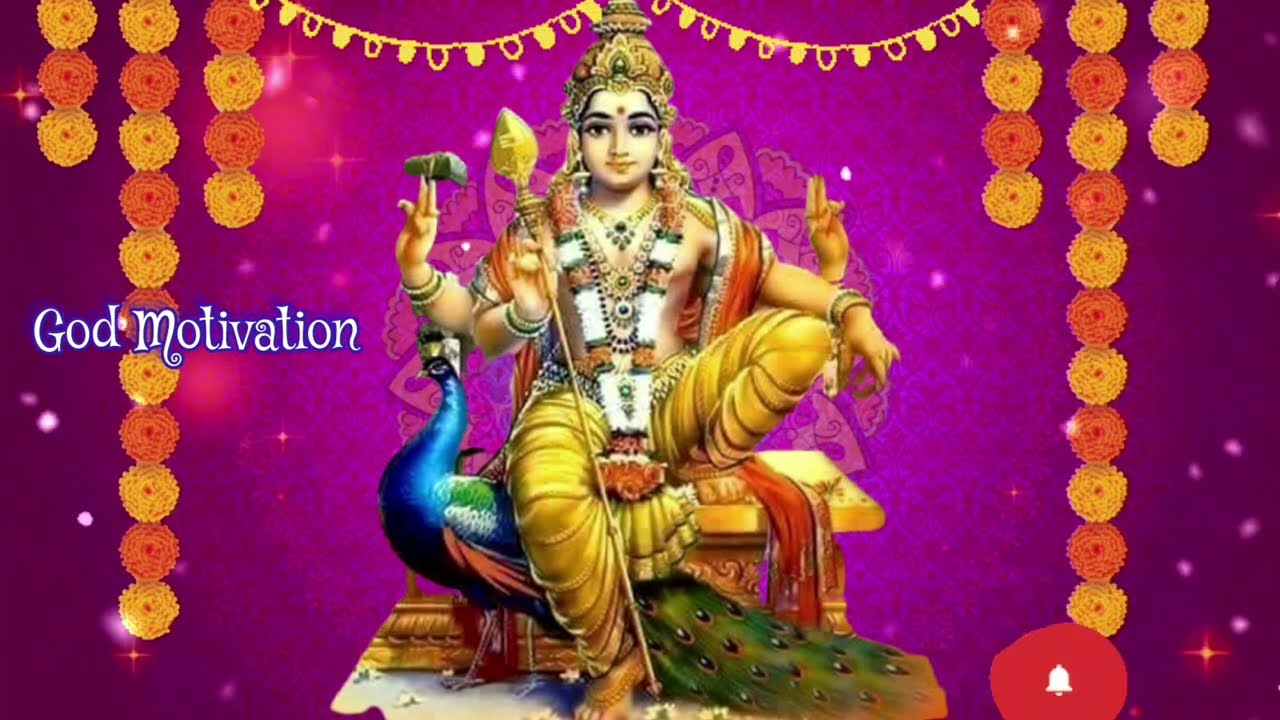The image depicts a detailed and vibrant illustration of a Hindu deity with four arms, seated on a golden stand. One leg is positioned with foot on the stand while the other rests on the ground. The deity, suggestive of a Buddha-like or East Indian divine figure, is adorned with a variety of elaborate accessories. The figure wears a large red, white, and black necklace extending down to the knee, along with another gold necklace featuring a black brooch. A crown ornate with golden embellishments sits on the figure's head, and there's a prominent red dot between thick, black eyebrows detailed with eye makeup. The lower part of the deity's attire comprises yellowish-golden pants and numerous bracelets. In its hands, the deity holds a golden rod and another green object, with two hands forming peace signs displaying different gestures. A vibrant peacock, hues of blue, green, orange, and red, stands beneath one of the legs. The background transitions from light to dark pink and purple towards the edges, embellished with sparkles and hanging ornaments, including red and orange round decorations resembling streamers and garlands draped elegantly. The words "God Motivation" are inscribed on the left side of the backdrop. The scene is heavily decorated, resembling a divine, artistic representation rather than a mere photograph.